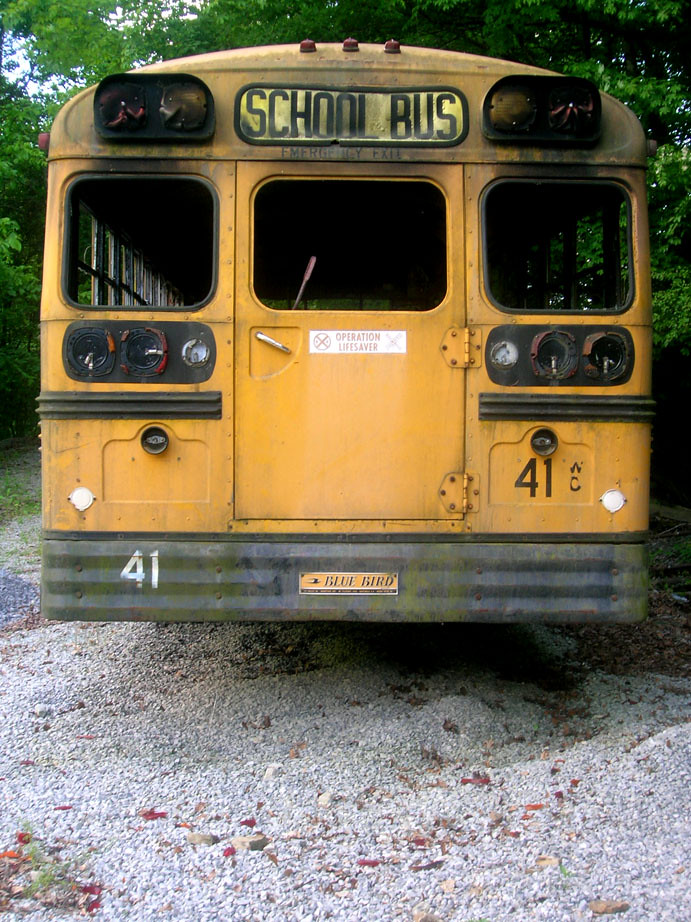The image depicts the rear view of an old, seemingly abandoned or partially burned school bus set amidst a natural backdrop of tall, green trees. The ground beneath the bus is scattered with light gray pebbles and red and brown fallen leaves. The bus, a standard yellow "Blue Bird" model, is faded, dirty, and slightly rusty. It bears signs of fire damage with black, smoke-like traces, particularly on the top and around the lights. The rear of the bus features a black fender with the number 41 displayed twice, once in white on the left and once in black on the right. The center of the fender has a yellow label with "Blue Bird" written in black. Above the rear door, which has a silver handle, "School Bus" is written in bold black letters on a yellow background, followed by "Emergency Exit" in black. A white sticker with red lettering reading "Operation Lifesaver" is prominently placed in the middle of the back door. The bus’s windows are broken, and the rear lights, including the taillights, are smashed and bent. The overall scene gives an impression of abandonment, with the bus nestled within the serene yet somewhat desolate natural environment.